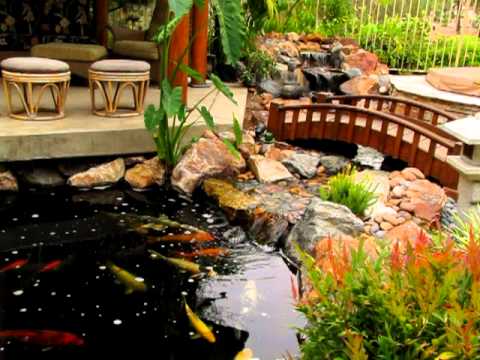This peaceful image depicts a serene water garden featuring a dark, pristine koi pond situated in the lower left corner. The pond is teeming with colorful koi fish, primarily in shades of yellow, red, and orange. Surrounding the pond are large, colorful rocks, and lush greenery, including wet plants accentuating the garden's tranquility. In the background, a small, arched red bridge gracefully spans the water, leading to a cascading waterfall that flows into the pond. This bridge is narrow, wide enough for only one or two people to walk across, and adds a picturesque element to the scene. On the upper left side of the image, a flat cement patio with two round, backless stools, ready for relaxation, provides a perfect spot for viewers to sit and admire the vibrant pond. Additional seating and two red columns frame the edge of the patio, enhancing the garden's inviting atmosphere. The overall composition exudes harmony and natural beauty, offering a tranquil retreat for contemplation.